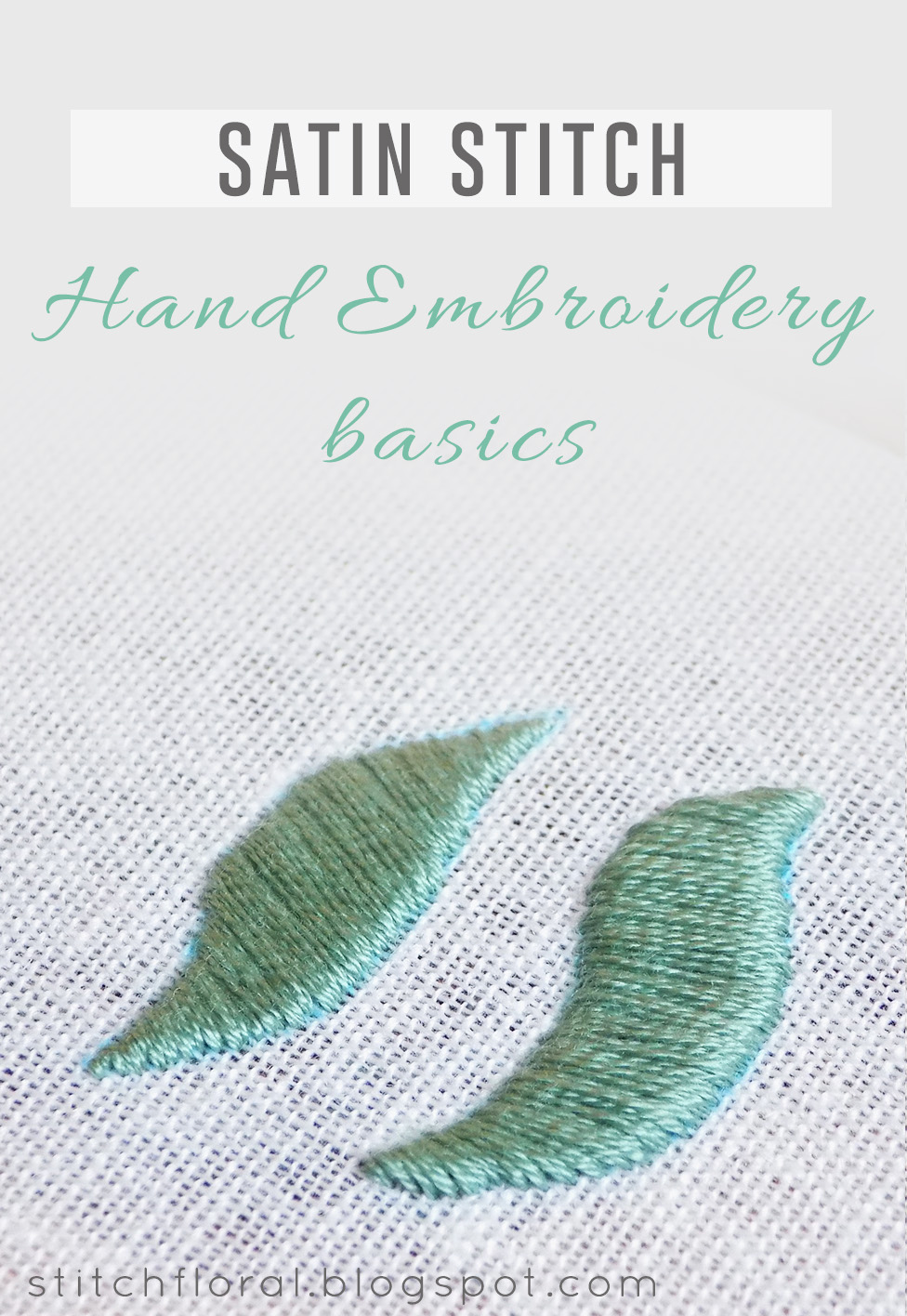The close-up image features a delicate piece of white cloth embroidered with two green, leaf-like shapes using satin green thread. The fabric, reminiscent of cheesecloth with visible individual threads, highlights the intricate hand embroidery. At the top of the image, a gray title in a white text box reads "Satin Stitchings," and beneath it, in green script font, it says "Hand Embroidery Basics." At the bottom of the fabric, text in a regular font reads "stitchfloral.blogspot.com."